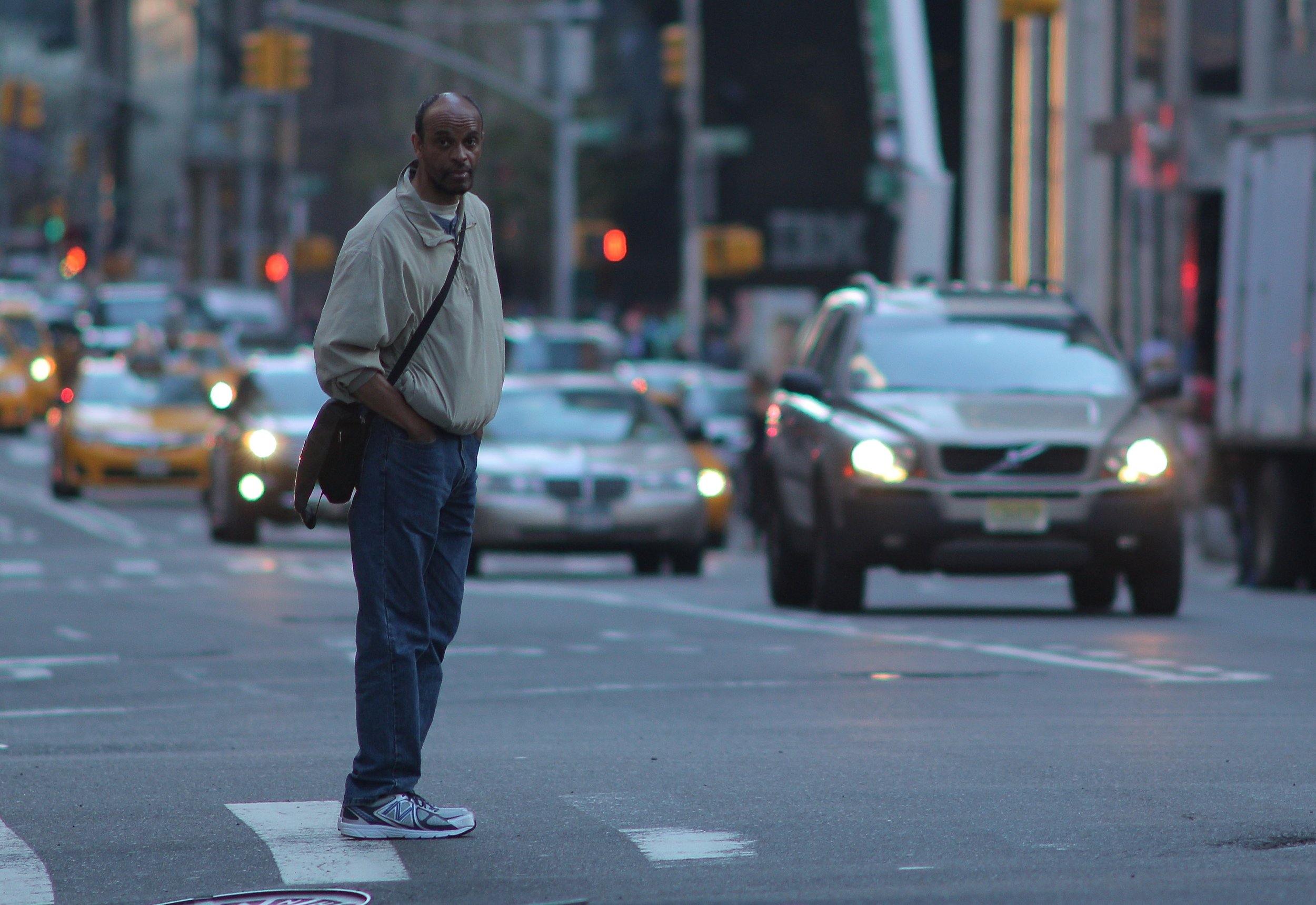In the heart of a bustling city, a tall, bald black man in his forties stands at the edge of a busy intersection, waiting to cross the street. He's positioned on the left side of the image, captured looking towards the oncoming traffic, which includes a mix of yellow taxis and various colored cars, all lined up and contributing to the rush hour chaos. He dons a tan windbreaker-style jacket with a zipper, layered over a blue Henley shirt and a white T-shirt. Blue denim jeans and blue-and-white sneakers complete his attire. Strapped across his left shoulder and resting on his right hip is a black satchel. With a darkening sky overhead and streetlights blinking on, he appears to have just finished his day, blending seamlessly into the urban landscape of towering buildings and crowded streets.